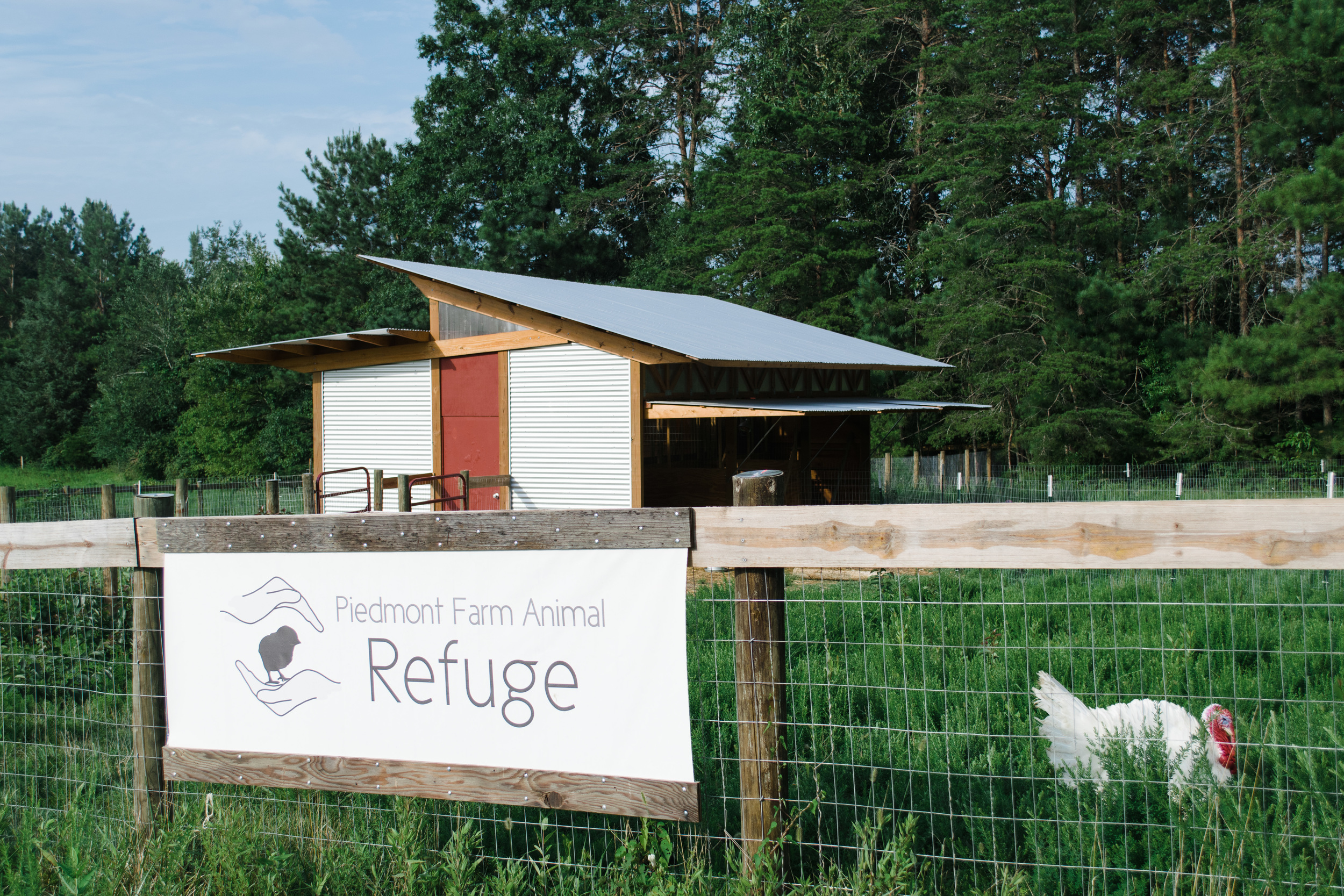The horizontal rectangular photograph depicts a serene scene at Piedmont Farm Animal Refuge on a sunny day. The central focus is a sign made of white wood with brown text and flanked by wooden posts, proclaiming "Piedmont Farm Animal Refuge." Above the text is a logo featuring two hands cradling a chick. This sign is positioned at the forefront of a wooden fence lined with wire, which encloses a lush, green field dotted with grassy patches and various trees.

In the background, a utilitarian building, possibly an animal shelter, stands prominent with its white walls, a closed red door, and multiple angled roofs in gray. There appears to be a garage-door-like front partially open, revealing a dark interior.

In the lower right corner of the image, a white turkey with a distinctive red neck stands on the green grass, adding a living, breathing element to the tranquil farm scene. The entire area is bathed in sunlight under a clear blue sky, emphasizing the vibrant greenery encompassing the refuge.